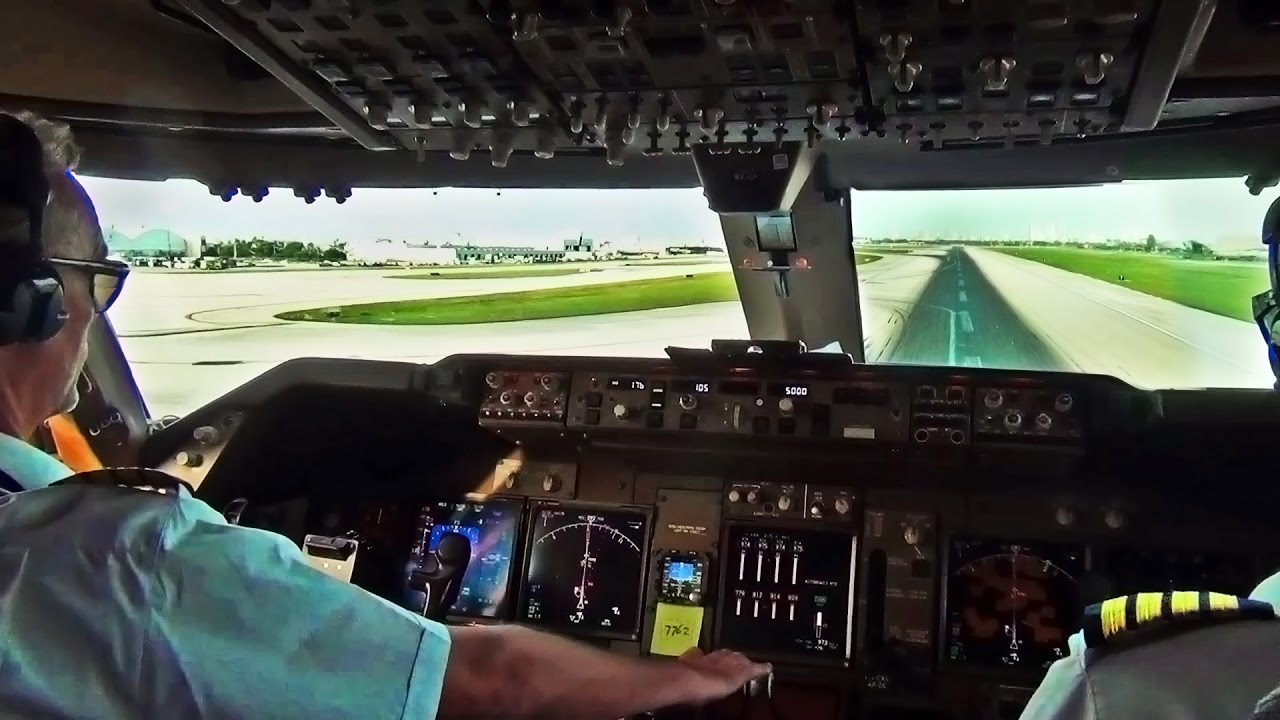In this detailed landscape layout photograph taken from inside the cockpit of an airplane, two pilots are visible side-by-side as they prepare for takeoff. The pilot on the left, identifiable by his glasses, gray hair, and headphones, is dressed in a blue short-sleeved button-down shirt with shoulder stripes and has his hand outstretched over an array of gauges, buttons, and knobs on the dashboard. The co-pilot, partially visible by his left shoulder, sports a matching uniform with a black label and gold stripes. Through the cockpit's windshield, the brightly lit runway with green grass borders and white stripes down the middle is clearly visible, indicating a sunny day. The cockpit itself is equipped with numerous controls, switches, and touchscreens essential for flying the plane.